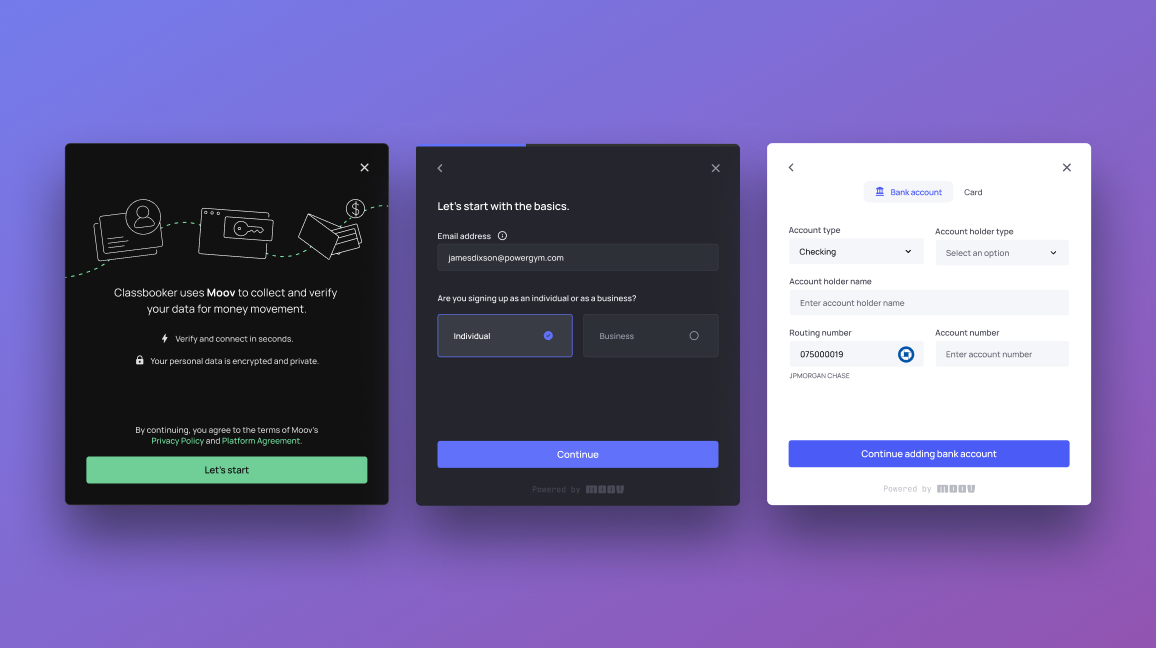Here is a cleaned-up and detailed caption for the image you described:

---

The image is a promotional graphic for a money management app, set against a large, vibrant purple background. It features three horizontally aligned screenshots showcasing the step-by-step process for connecting accounts and tracking spending. 

The **first screenshot** on the left displays the app's main page. At the bottom, there is a prominent green button labeled "Let's Start." The page contains descriptive text detailing the app's functionality, mentioning how "Class Blocker uses Move to collect and verify your data for money management."

The **second screenshot** in the middle introduces the initial setup screen, titled "Let's Start with the Basics." It features an input field for an email address, options to sign up as an "Individual" or "Business," and a blue "Continue" button at the bottom.

The **third screenshot** on the right focuses on the account connection interface. Two tabs labeled "Bank Account" and "Credit Card" are displayed, with "Bank Account" being selected. The screenshot shows input fields for entering bank account details, concluding with a blue button at the bottom that reads "Continue Adding Bank Account."

Each screenshot is neatly centered on the purple background, providing a clear and organized visual guide for new users setting up their accounts.

---